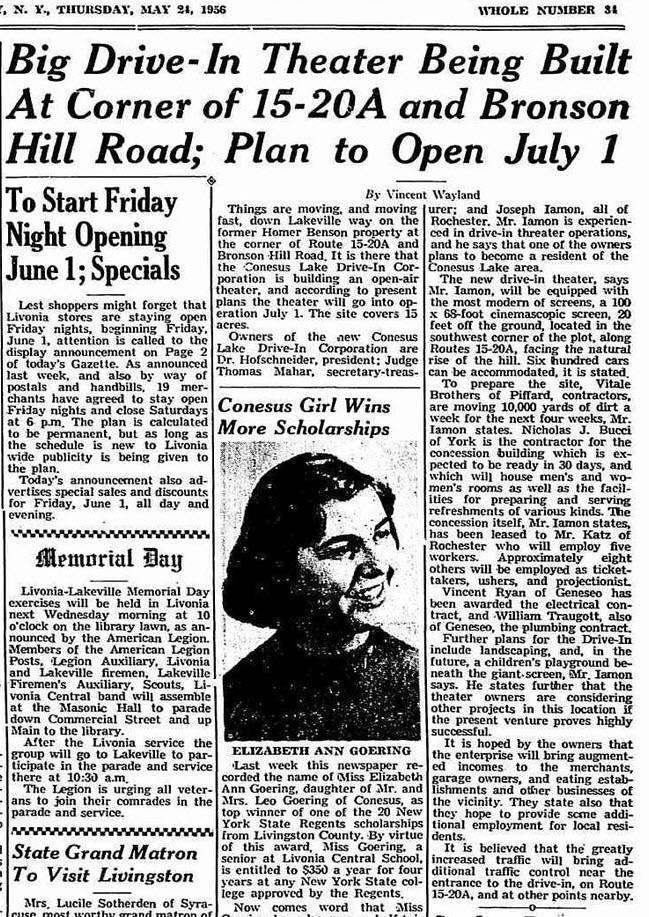This image captures a vintage newspaper clipping dated Thursday, May 24, 1956, from page 34. At the top, the headline announces a "Big Drive-In Theater being built at the corner of 15 F and 20 A and Bronson Hill Road, planned to open July 1." Below this, there is a smaller title mentioning "To start Friday night, opening June 1 specials." The page is sectioned off with black lines and squares labeled "Memorial Day," followed by two to three detailed paragraphs.

In the central segment, the article "Consensus Girl Wins More Scholarships" features a black-and-white headshot of Elizabeth Ann Goring. She is posed with her head turned to the right, displaying her dark, short, shoulder-length hair and a dark top. Her picture is a prominent element of the page. 

To the right of her photo, another article by Vincent Wayland appears, fully filling the column with text. Lower on the page, another headline reads, "State Grand Matron to Visit Livingston." This full page of articles and announcements is completely in black and white, capturing the essence of a mid-20th-century newspaper.